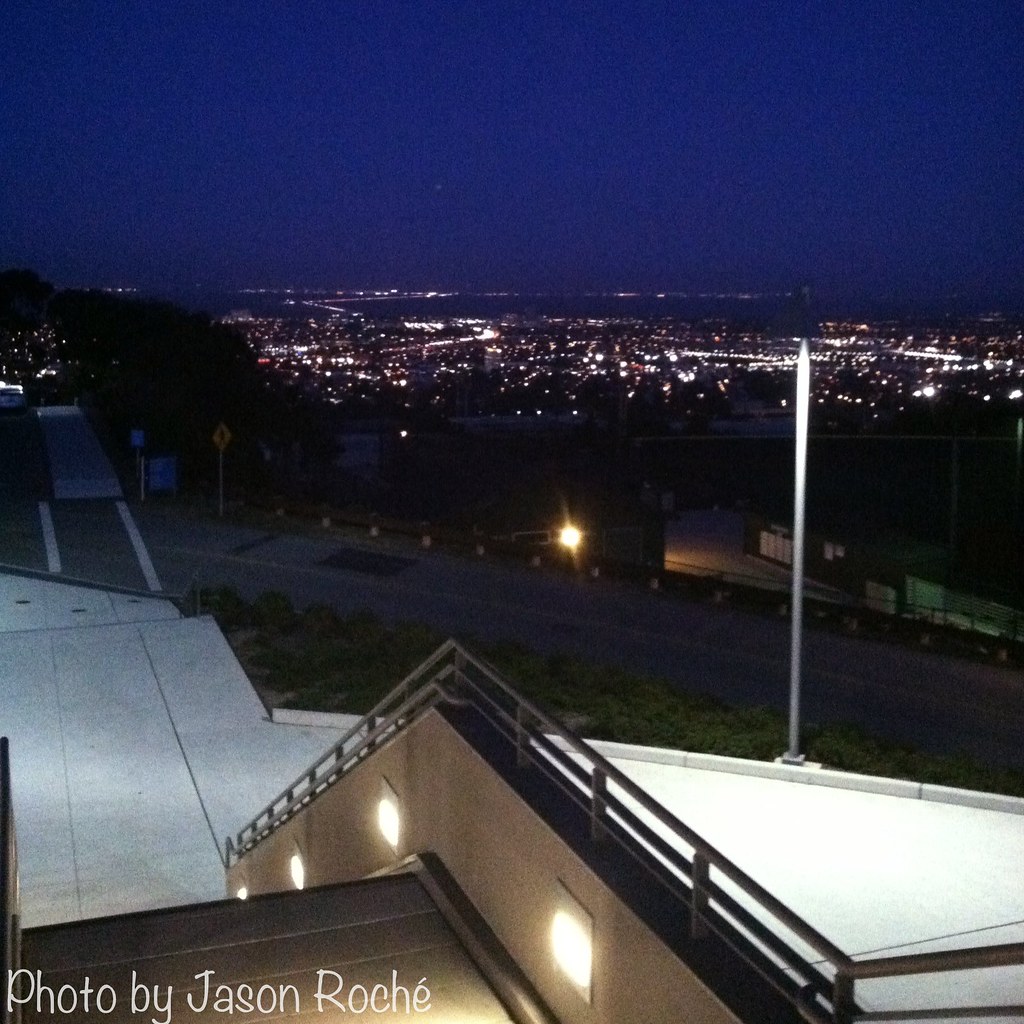This nighttime photograph, credited to Jason Roche in white text at the bottom left corner, captures an expansive cityscape seen from an elevated vantage point, possibly a balcony or rooftop. The foreground features a well-lit, descending staircase with gray-brown steps and a small chair, suggesting it was taken "up in the air" looking down. Below, several houses with slanted roofs—some adorned with white lights and brown panels—are visible. In front of the houses, a two-lane road with a double yellow line is accompanied by patches of greenery. The background reveals a sprawling city illuminated with a myriad of lights against a dark blue sky, highlighting the bright, bustling life of the city at night.